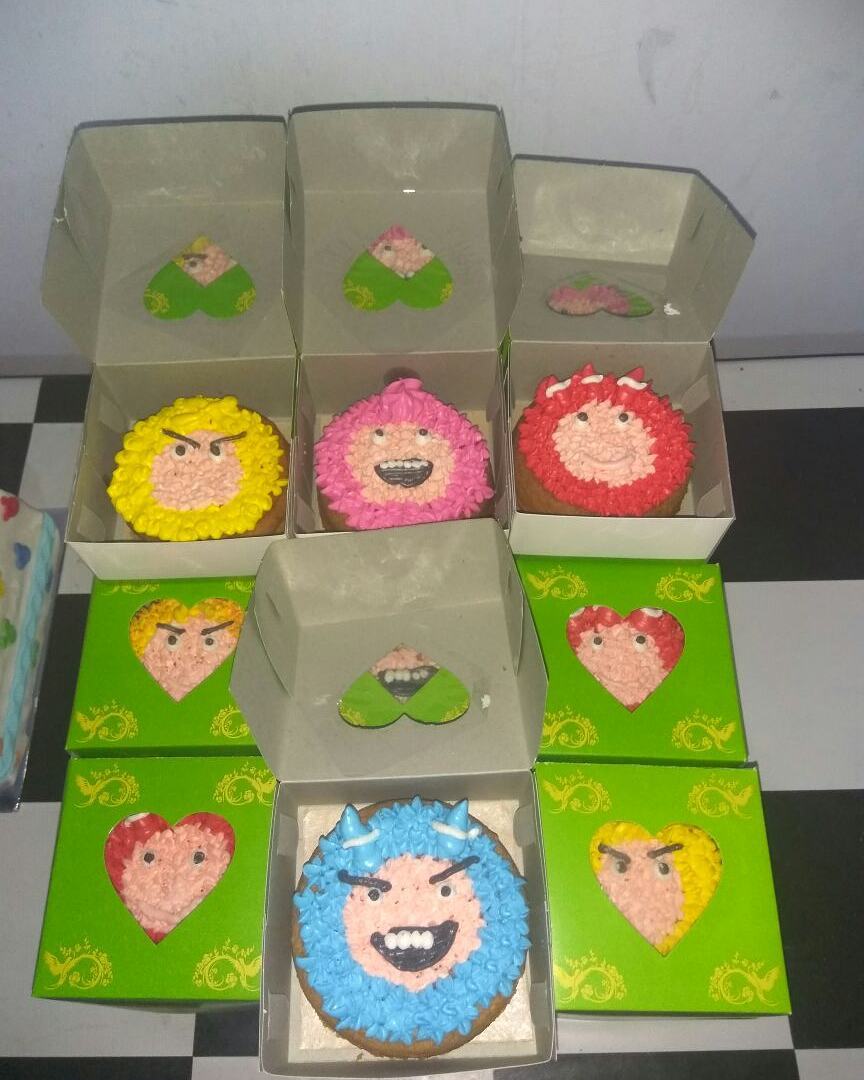This vibrant portrait-oriented photograph showcases nine custom cupcakes, each with a distinct face and colorful frosting, inside green boxes adorned with yellow drawings. At the center of each box is a heart-shaped, see-through window that reveals the playful expressions of the cakes within. Four of the boxes are open, showcasing their whimsical designs in more detail. One cake, with yellow frosting, features eyes and eyebrows with an incomplete face. Another cupcake, enveloped in pink frosting, displays a cheerful smile with its eyes looking upward. The third visible cake, bathed in red frosting, presents a subtle smile with eyes glancing sideways. The fourth, positioned prominently at the bottom, is striking with blue frosting and sports black horns along with a black-lipped, toothy grin and eyebrows. These enticing cakes, likely chocolate, exhibit a unique and delightful variety, making them perfect for showcasing on a website or as a custom-made treat. The photograph, devoid of any text, focuses purely on the visual appeal of these quirky, expressive cupcakes, each nestled in their uniformly green, creatively designed boxes.